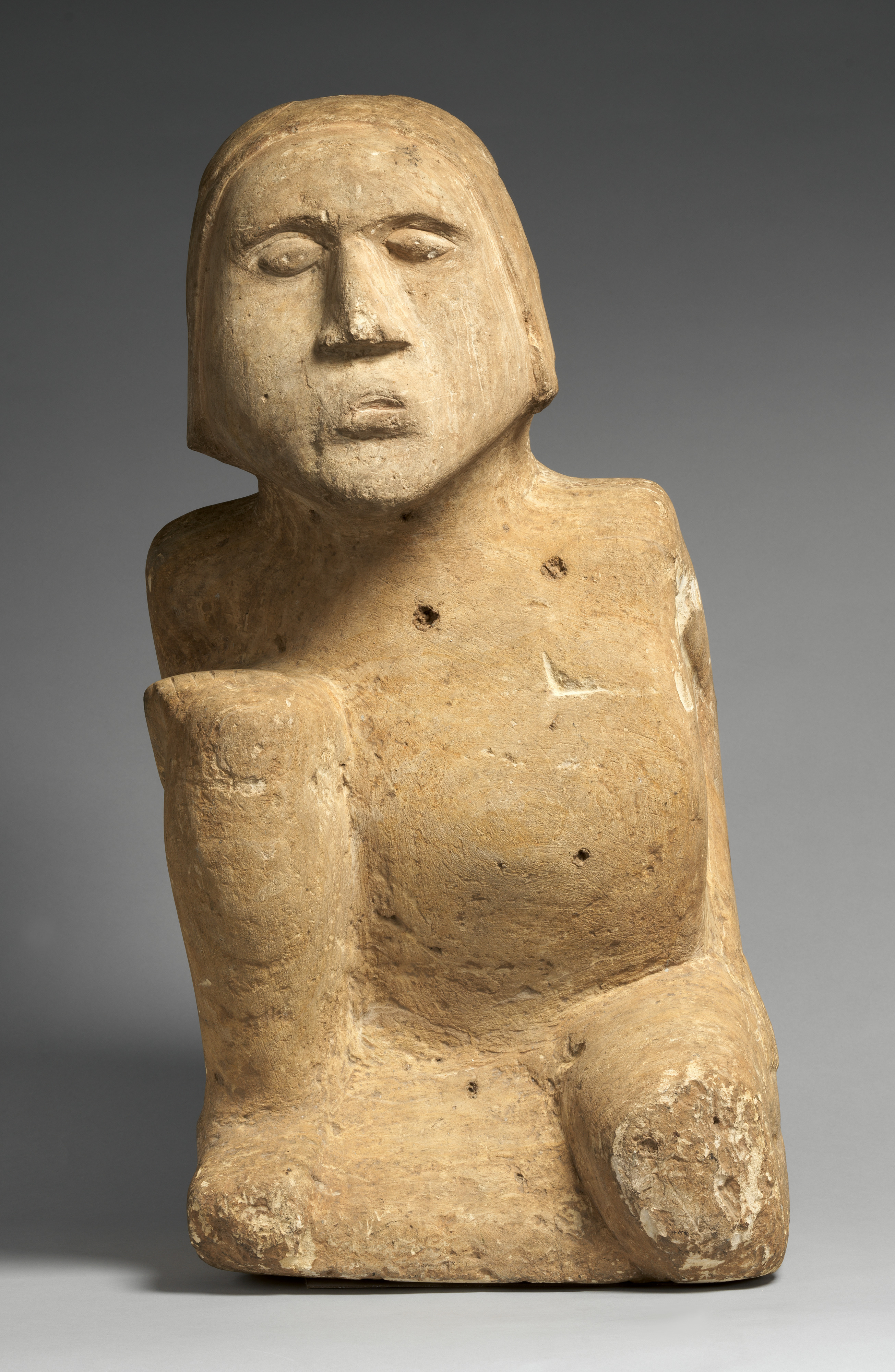The image showcases an antique, light brown stone statue set against a neutral gray backdrop. Depicting a person likely intended to be male, the statue is remarkably old and shows significant signs of wear. The figure has a broad nose, short chin-length hair, a small mouth, and eyes that appear closed with long eyelashes, although the pupils are barely visible due to erosion over time. The torso of the statue is intact but entirely lacks arms and legs, with fragmented remains hinting at their former presence. Particularly on the right side, what seems to be a partial leg abruptly ends, suggesting breakage. Additionally, a distinctive, thick cylindrical piece rises on the viewer's left side, though its purpose and connectivity to the statue remain unclear. The stone surface is pocked with numerous holes, enhancing its ancient and weathered appearance.